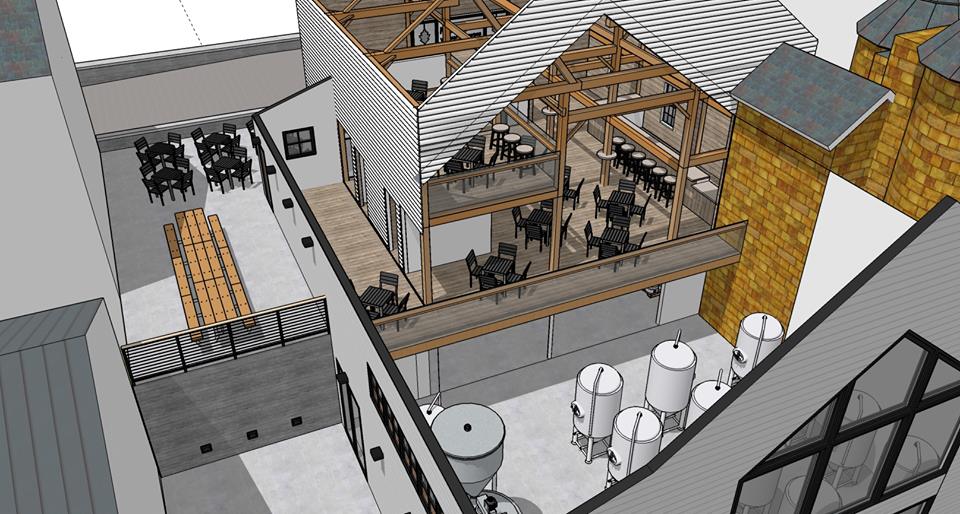This is a detailed, cartoony illustration of a restaurant viewed from above, with the roof removed for an interior view. The building's walls are white with brick columns on the left side. The layout reveals multiple dining sections: in the back left corner, an outdoor deck area features a room with a brown motif, including four round tables with chairs and a long rectangular table with benches. Further towards the center and right, the restaurant extends over two levels. The lower level contains several black square tables, each surrounded by four matching chairs and accompanied by a bar area with black bar stools. Below the dining area, arranged on a concrete floor, are six white containers resembling fuel tanks or silos, likely used for storing beer or wine. The color scheme predominantly features grey and brown tones, with black furniture accentuating the dining spaces. The restaurant's open design and diverse seating arrangement suggest a vibrant dining atmosphere.